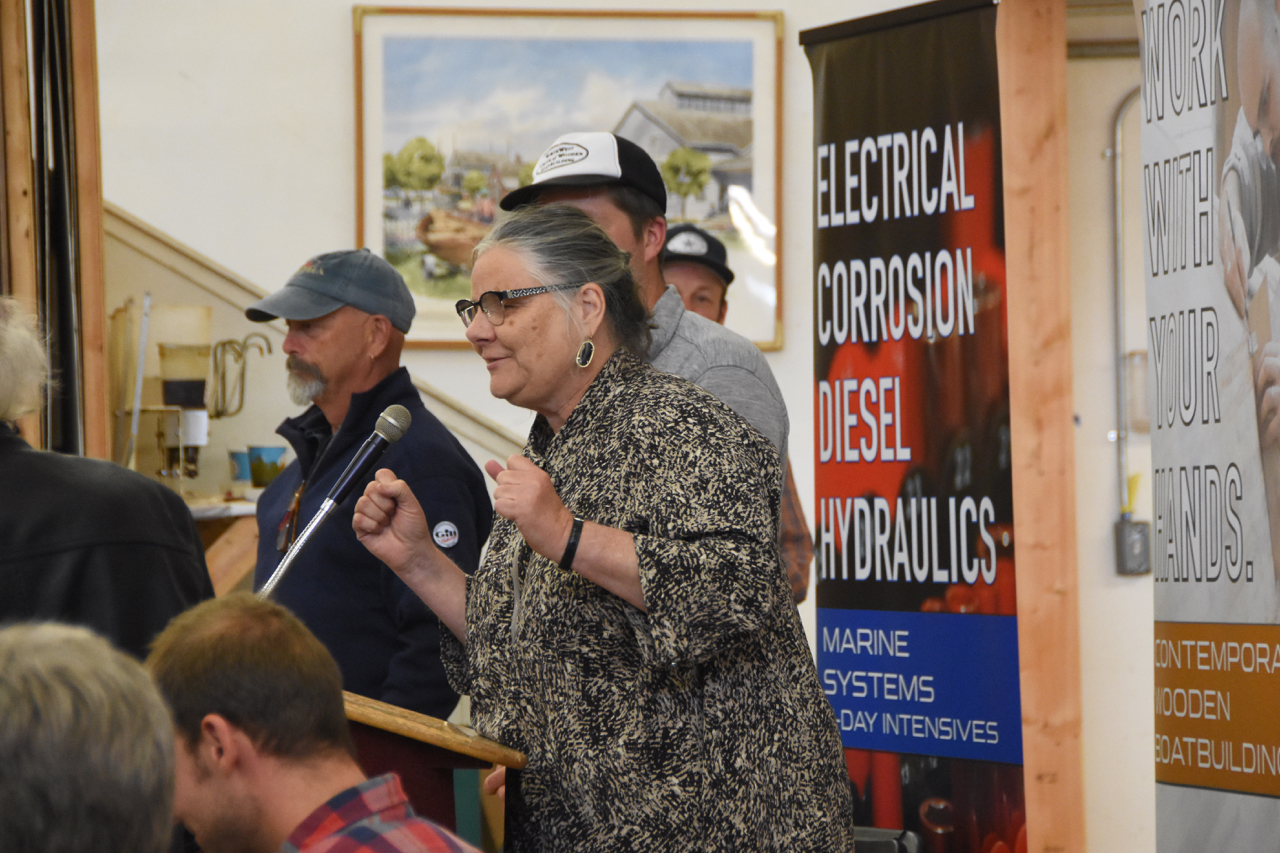In this image, an older woman is depicted standing behind a podium while speaking into a microphone that is positioned close to her face. She is wearing a distinctive black and gold shirt and has gray hair and black glasses, which add a sense of wisdom and authority to her presence. She appears to be addressing a gathering, as there are several people surrounding her, attentively listening to what she has to say. 

Beneath the podium, there are two prominent signs. The first sign, positioned to the left side of the image, lists various technical disciplines such as electrical corrosion, diesel, hydraulics, and marine systems. It also mentions "day intensives," indicating a focus on concentrated learning sessions. The second sign, located on the right-hand side of the image, encourages a hands-on approach to learning with phrases including "work with your hands" and "contemporary wooden boat building." 

Despite the informative context provided by the signs, the woman at the podium is the focal point of the image, suggesting she is likely an expert or key speaker at this event, contributing valuable insight on the subjects mentioned.